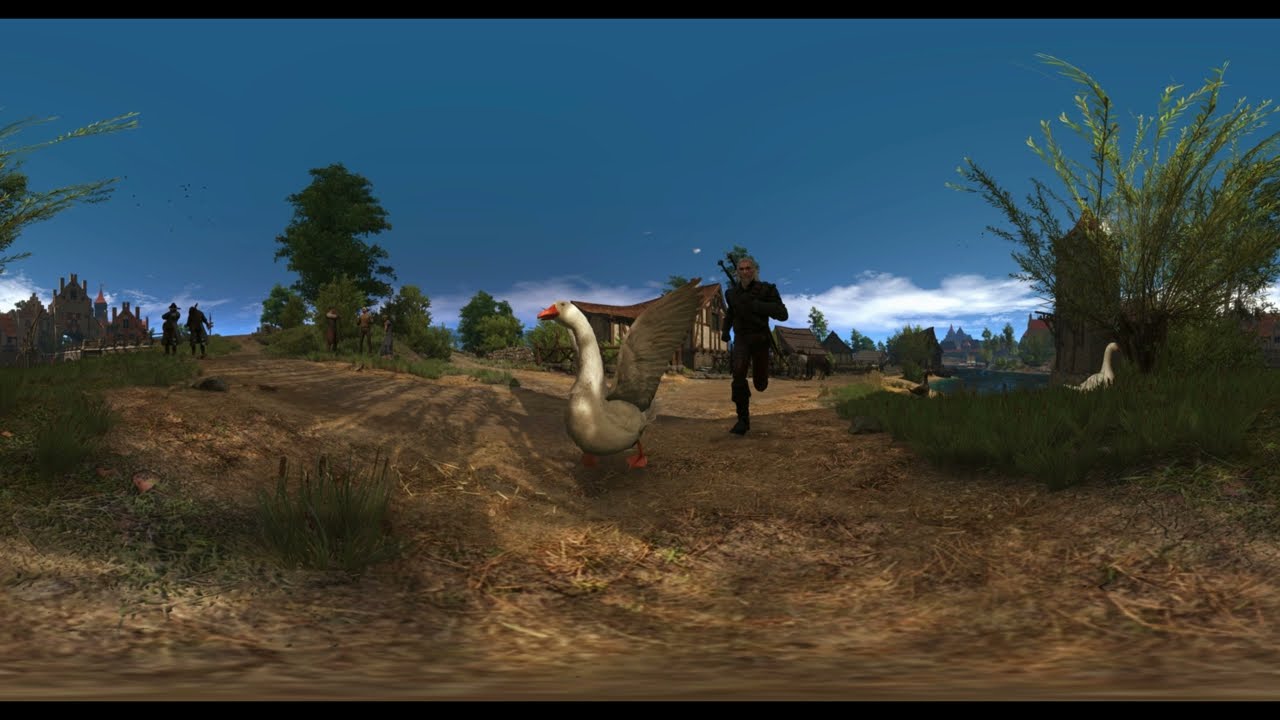The image, a screenshot from a video game, captures a lively scene set on a dirt path with patches of straw and green grass, flanked by lush green trees that suggest a summer setting. At the center, a man dressed in black and carrying a sword is running toward the camera, chasing a white goose with its wings extended. Off to the right, another goose wanders among shrubs and bushes. The background reveals a European-style village with a two-story house and smaller outbuildings, as well as a larger, castle-like building further in the distance. The sky is a bright blue, adorned with a few white clouds. Adding to the depth of the scene, two people are seen conversing on the left side of the path. A thin black bar runs horizontally across the top and bottom of the screen, framing the image.